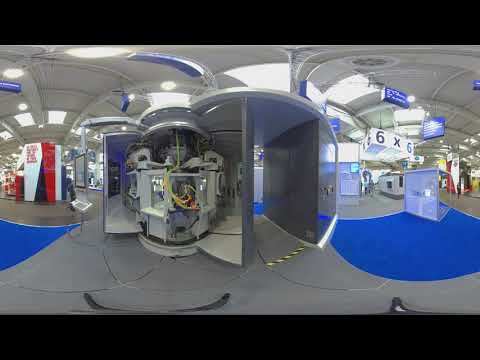The image depicts an industrial showroom interior with a vaulted white ceiling adorned with curved pipes. Numerous brown signs hang from the ceiling, and the gray floor features round blue patterns. On the left side, there is a rectangular booth with a white and red cover. The centerpiece is a gray machine emitting blue and red lights, with intricate wiring and mechanical components, including a cylindrical space that appears accessible and an adjacent pillar. To the right, white signs displaying "six times six" are suspended overhead. The space, captured in a panoramic view, is well-lit and official, characterized by heavy machinery, blue markers, and caution tape on the floor, enhancing its industrial aesthetic.